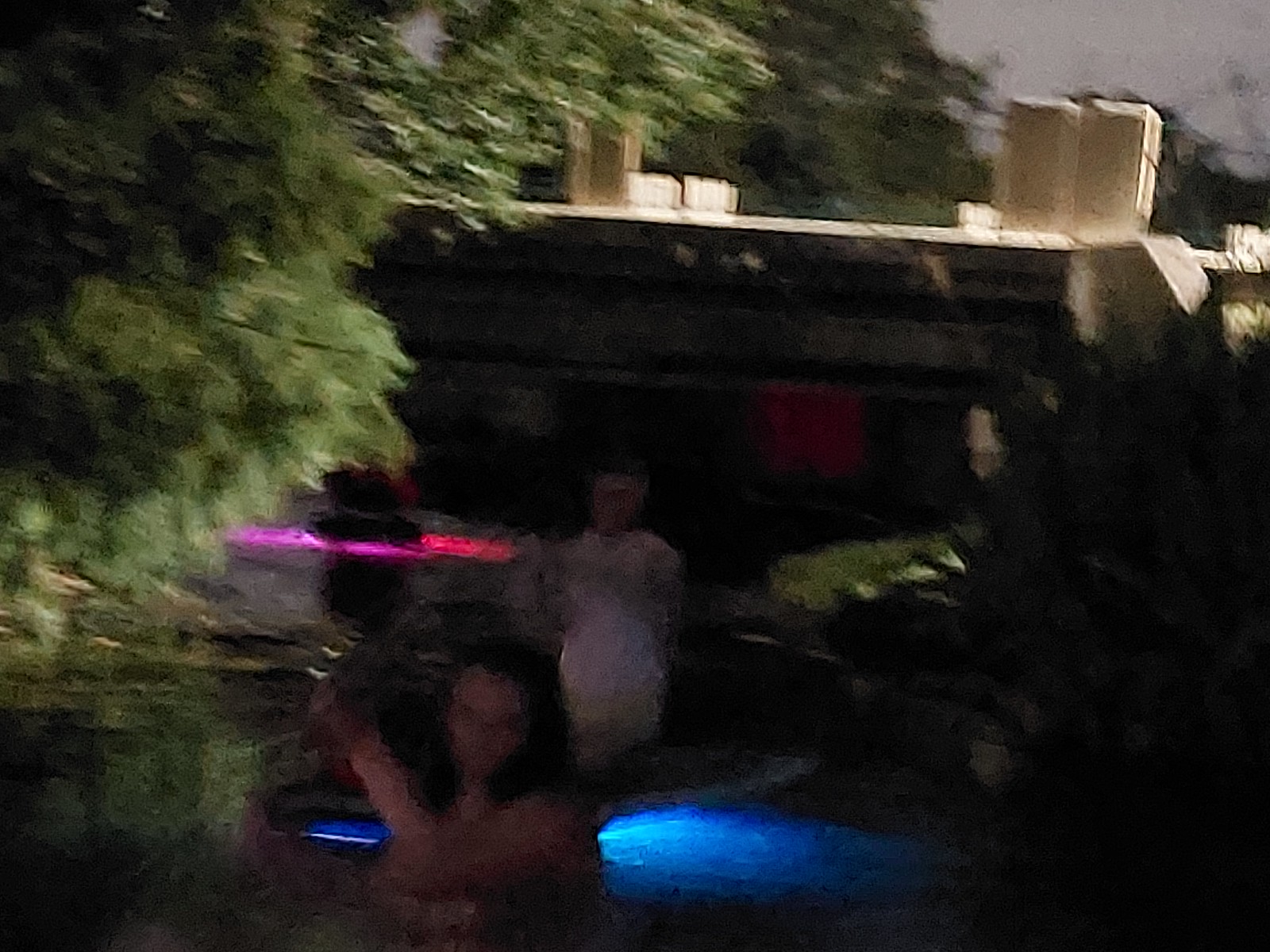Amidst the dim, nocturnal ambiance, a blurred photograph captures two women standing in what appears to be a porch or pool area. The younger woman in the foreground has dark hair and a fair complexion, and is dressed in a bathing suit or a thin-strapped top. She holds an unidentified object above her hand, surrounded by a captivating halo of pink and red light, possibly a drone. Behind her stands an older woman, wearing a light-colored shirt and yellow pants, observing the younger woman's actions. A blue glow between them hints at water or ambient outdoor lighting, adding to the enigmatic atmosphere. The backdrop includes the roofline of a house and dark, dusky sky, with woods and foliage visible to the left, reflecting subtly in what might be water. The top right corner of the image reveals a glimpse of the night sky, completing this mysterious, multi-layered scene.